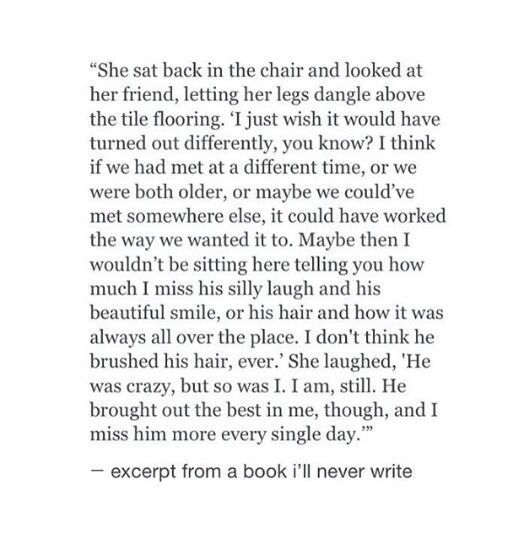The image portrays a poignant passage from a book, titled anonymously as "Excerpt from a book I'll never write," in simple black and white text. The passage reads: "She sat back in the chair and looked at her friend, letting her legs dangle above the tile flooring. 'I just wish it would have turned out differently, you know? I think if we had met at a different time or we were both older, or maybe we could have met somewhere else, it could have worked the way we wanted it to. Maybe then I wouldn't be sitting here telling you how much I miss his silly laugh and his beautiful smile, or his hair and how it was always all over the place. I don't think he brushed his hair ever,' she laughed. 'He was crazy, but so was I. I am still. He brought out the best in me, though, and I miss him more every single day.'" The excerpt captures a reflective and bittersweet nostalgic conversation about a past lover, set against a minimalist backdrop, emphasizing the emotional weight of the words.